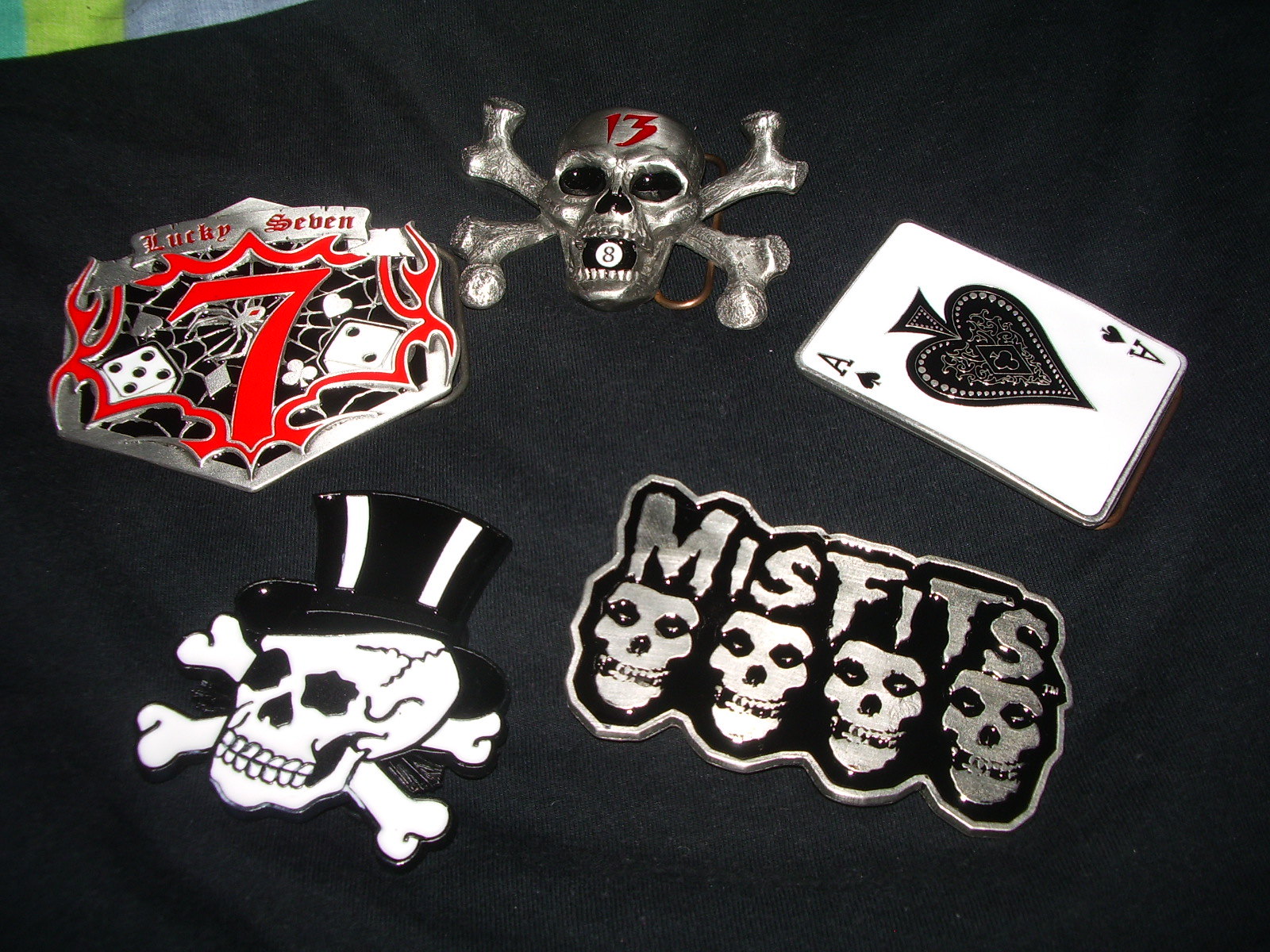The image features a neatly arranged collection of distinct metal pins displayed on a black tablecloth. Among the five items, there's a striking white Ace of Spades card pin, prominently showcasing its bold black emblem. Another pin features an intricate design of a skull and crossbones with a black and white top hat, while a second skull and crossbones pin made of silver has a red number "13" emblazoned on its forehead and an open mouth displaying the number "8." Additionally, a large red "7" stands out on a pin labeled "Lucky 7," which includes a spiderweb background and a pair of black and white dice, one showing "5" and the other "2." The final piece in the collection is a silver artwork with the word "Misfits" at the top and a quartet of eyeless skulls at the base, completing the gothic and eclectic ensemble.